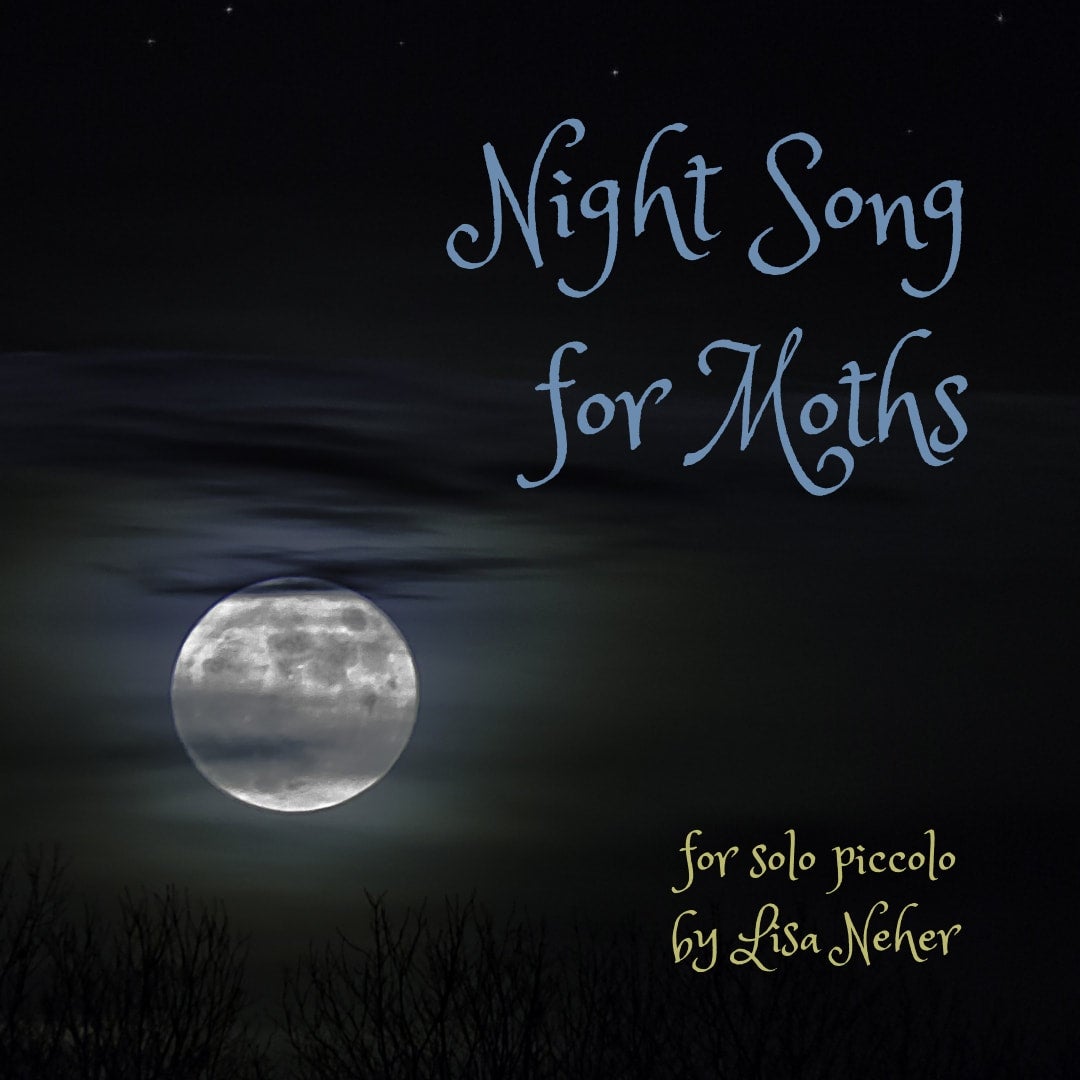This image, likely an album cover, presents "Night Song for Moths" in blue lettering, positioned towards the center right. The artist’s name, Lisa Neher (N-E-H-E-R), is written in smaller, yellow font at the bottom right of the cover, with the piece specifically designated as "For Solo Piccolo." The background is a black night sky, punctuated by a few stars at the top edge. Dominating the scene is a large, white full moon with visible craters and thin, wispy clouds drifting across it. This moonlight reveals the faint silhouette of barren branches and a hint of tundra landscape below. The overall composition, blending natural and celestial elements, evokes a mystical nocturnal atmosphere.